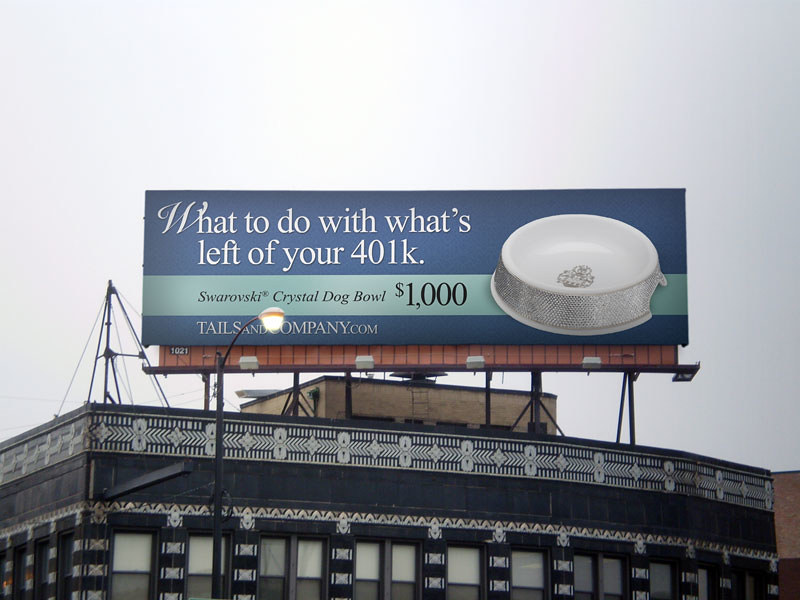The photograph captures the top of a flat-roofed building adorned with a large horizontal rectangular billboard. The sky behind the structure is overcast, presenting a gradient from white at the center to shades of gray and gray-blue at the edges, contributing to a hazy atmosphere.

The prominent billboard, set against a dark blue background, features the following text in bold statement:

1. "What to do with what's left of your 401K" at the top.
2. Below that, on a light blue band, it reads "SWAROVSKI Crystal Dog Bowl, $1,000."

Under this, again on the dark blue background, is the website address "tailsandcompany.com". 

An image of the advertised dog bowl, which appears to be white enamel with crystal embellishments along its edge, is displayed. Though there is some writing inside the bowl, it is not legible from this vantage point.

The building itself is dark gray and has a distinctive decorative tiling along its edge, arranged in a chevron pattern. The lower portion of the building reveals a glimpse of windows, adding a structural context to the image.